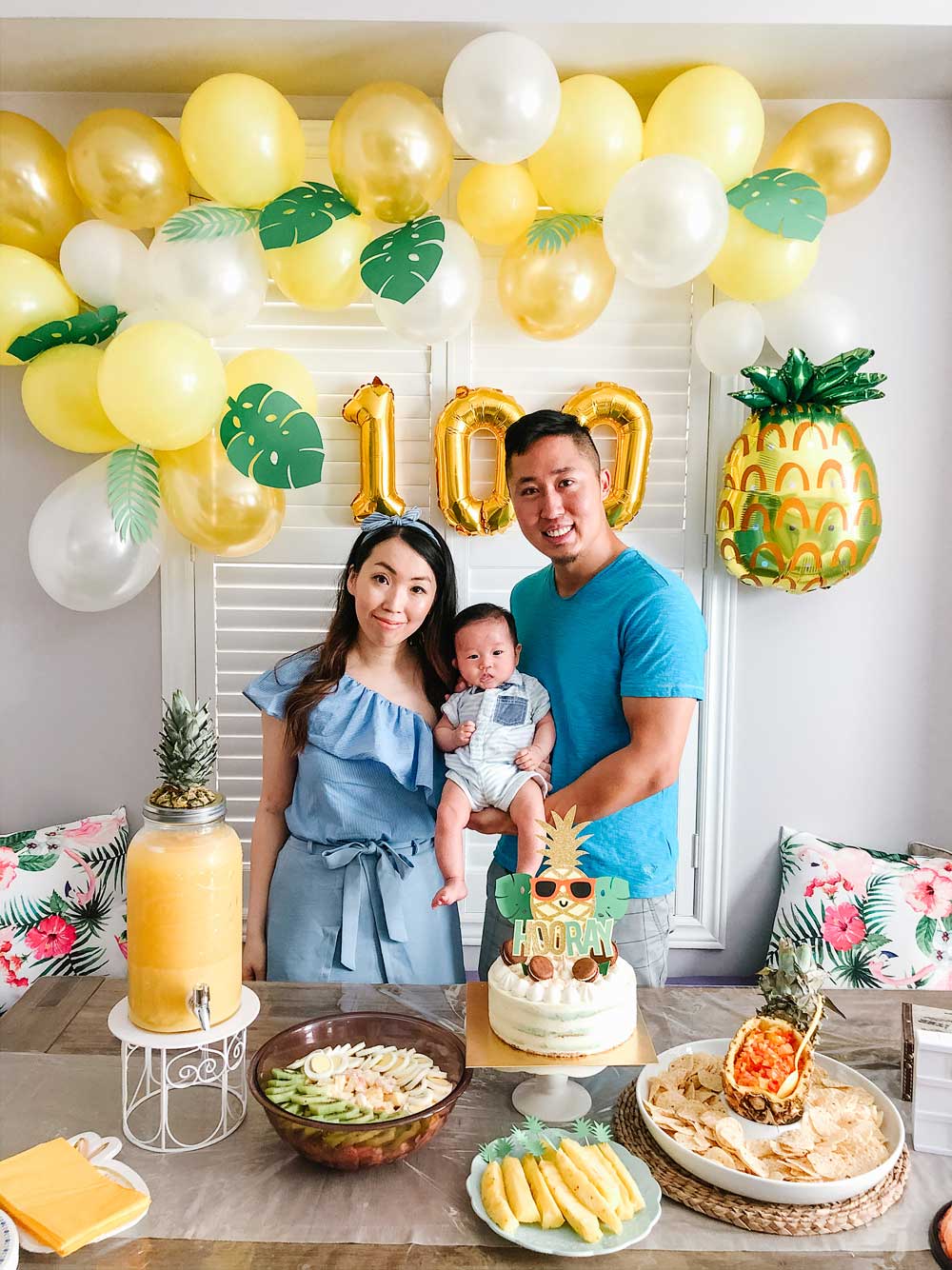In this vibrant birthday party scene, a beaming couple stands proudly with their baby. On the left, the woman, with her long dark hair adorned with a bow, is dressed in a light blue dress. The man on the right, sporting a turquoise blue shirt, holds their baby in his buff arm. The baby, nestled between them, is donning a light blue striped white onesie with short dark hair and bare legs. 

On the table in front of the family, a festive white cake bearing the word "Hooray" and decorated with a pineapple wearing sunglasses stands out, flanked by various tropical-themed items. Surrounding the cake are a platter of pineapple-tipped skewers, a cut pineapple bowl filled with salsa accompanied by chips in a white dish, and a clear bowl containing slices of egg, chicken, and kiwi. Additionally, there’s a jug of pineapple juice topped with a pineapple head. 

Above them, the backdrop features a cheerful arrangement of yellow and white balloons and the number "100" in large balloon figures, adding a celebratory touch to the scene.